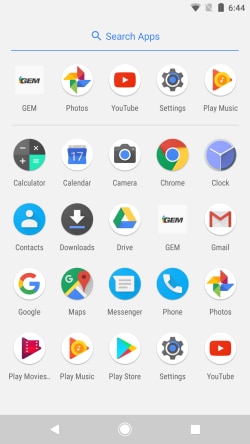The image depicts a smartphone screen showcasing various app icons arranged in a grid layout against a grayish-white background. At the top of the screen, there is a status bar that includes a Wi-Fi signal icon, battery indicator, and the time "6:44." Below the status bar, a blue line separates the interface from the search bar, which reads "Search apps" accompanied by a magnifying glass icon pointing to the left.

The apps are organized in rows as follows:

- First row: Gym, Photos, YouTube, Settings, Play Music
- Second row: Calculator, Calendar, Camera, Chrome, Clock
- Third row: Contacts, Downloads, Drive, Gym, Gmail
- Fourth row: Google, Maps, Messenger, Phone, Photos
- Fifth row: Play Movies, Play Music, Play Store, Settings, YouTube

Each app is represented by a distinctive and colorful icon. For example, the Google Chrome app is marked by its iconic multicolored circular symbol, while the Phone app is represented by a white phone icon set inside a blue circle. The overall design is orderly and ensures that each app is easily identifiable by its unique symbol and color scheme.